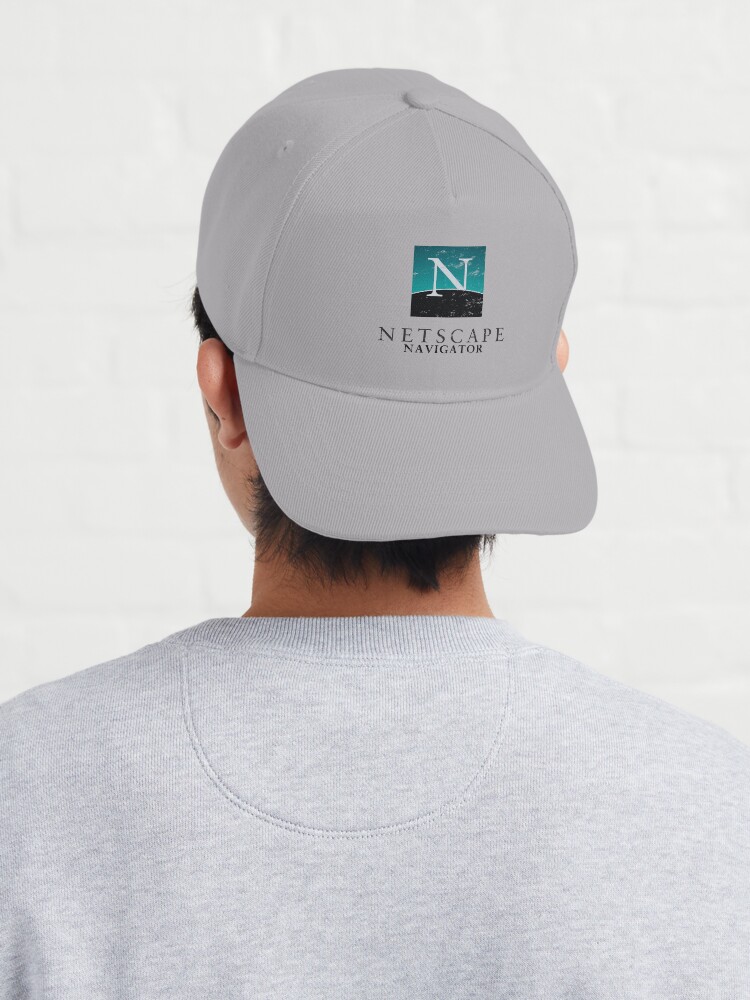The image showcases a young individual, likely hipster, with short dark hair and a Caucasian neck, donning a backward gray baseball cap. The cap prominently features a teal and blue square logo with a white "N" inside it, possibly representing a night sky or mountain scene, and bears the inscription "Netscape Navigator" in black below the logo. The person is seen from behind against an off-white, brick-like background, and is also wearing a gray heather sweater with a distinct circular neckline pattern that extends down their back. The scene emphasizes the person's casual, modern style while highlighting the detailed design elements of the hat.